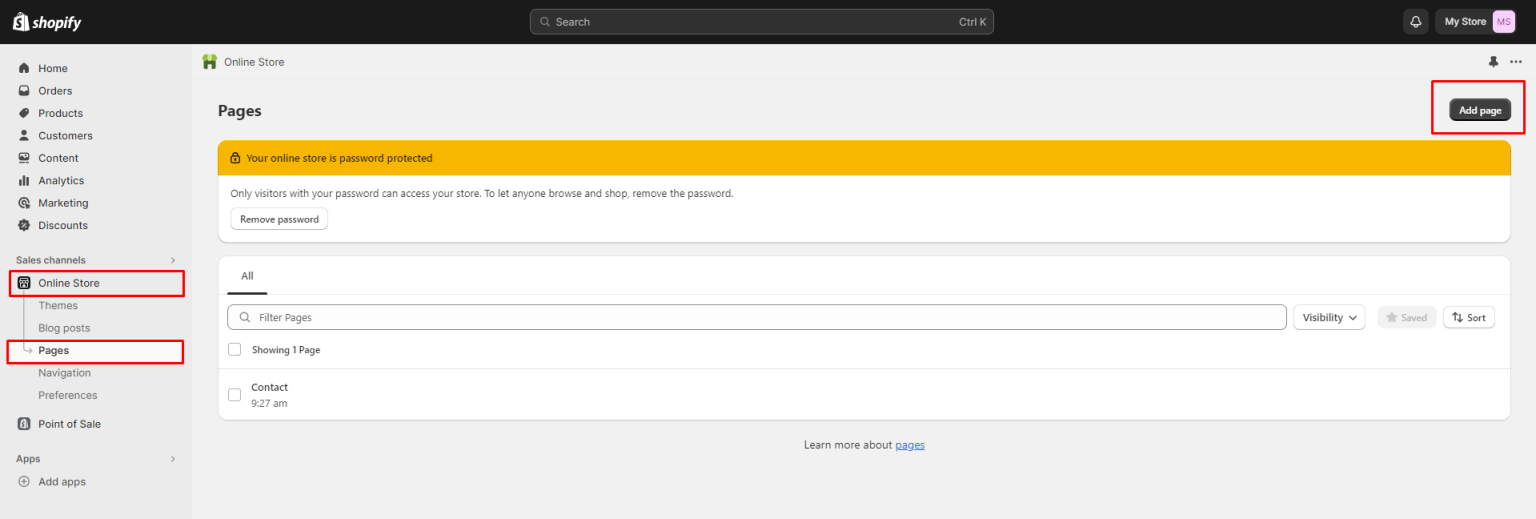This is a close-up screenshot highlighting various elements of the Shopify user interface at 200% zoom. At the top, there is a black bar, below which resides a gray search bar. To the right of the search bar, it displays "My Store" and "Online Store." On the left side, there is a vertical navigation column listing several options: Home, Orders, Products, Customers, Content, Analytics, Marketing, Discounts, Sales Channels (with "Online Store" highlighted in red), Themes, Blog Posts, Pages (highlighted in white and surrounded by red), Navigation, Preferences, Point of Sale, and Add Apps. Below the navigation column, a message indicates "Your online store is password protected," explaining that only visitors with the password can access the store and instructing users to remove the password to allow browsing and shopping. Further down, the "Pages" section is visible with a filter option and listings such as "Contact" under "All" with additional details about the store's password protection repeated at the top of this section.